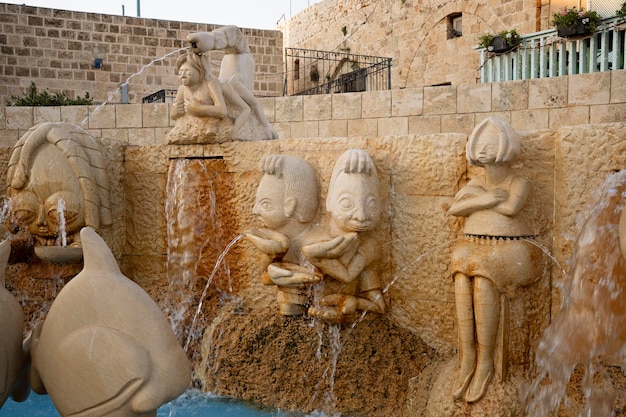In this whimsical outdoor sculpture garden, a variety of playful, larger-than-life stone figures function as water fountains, each uniquely designed to channel water in different ways. Dominating the scene are two humanoid sculptures with disproportionately large heads; one appears to be spewing water from its mouth into its hand, while the other features water streaming from its eyes. Another prominent figure is a woman with water flowing from her waist. Adding to the eclectic mix, there is a figure resembling a large whale and one that might be a fancy tortoise head. These sculptures, characterized by their light brown stone color, are set against a backdrop of intricate stone walls in various shades of tan and brown. The walls feature additional water spouts and are complemented by sections of wrought iron and white picket-looking fences adorned with hanging planters brimming with green plants. In the distance, a tan and brown brick building with balconies and wrought iron details enhances the picturesque setting.